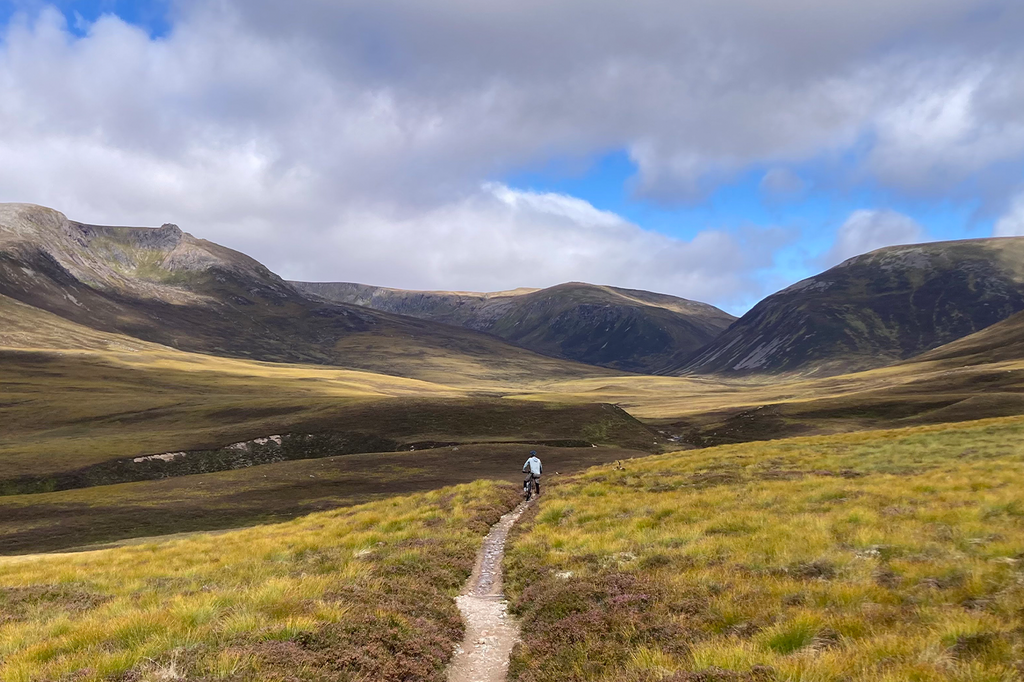This color photograph, taken in landscape orientation, captures a lone mountain biker riding along a narrow dirt trail that winds through a picturesque valley. The biker, dressed in a white top and wearing a black helmet, is seen from behind, positioned slightly to the lower center of the image as he gazes ahead. The trail itself, a mix of dirt and gravel, stretches from the foreground up into the distance, where it disappears over a hill on the horizon. 

On either side of the path, the grass is a blend of green and yellow hues, dotted with patches of light green hills and various weeds. Further into the background, the valley opens up into a vast prairie covered in beige-colored grass, bordered on one side by a small, dark brown stream partially obscured by trees. The distant landscape is dominated by rising mountains, their peaks shrouded in shadows and light gray rock, adding to the rugged beauty of the scene. Above, the sky is a mix of blue and the encroaching presence of ominous white and gray clouds, suggesting an impending change in weather. The overall style of the photograph can be described as Photographic Representationalism Realism, reminiscent of a freeze frame from a GoPro video, providing a dynamic and immersive view of the solitary biker's journey through this expansive natural setting.